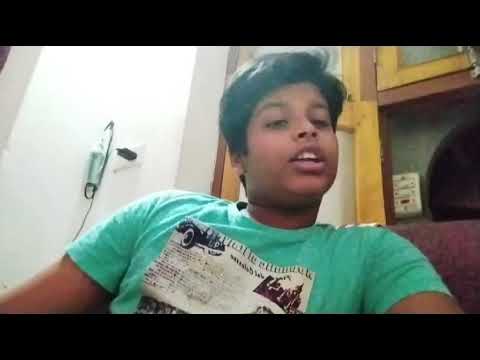This is a detailed photo of a young boy, likely around 12 years old, with dark, thick hair that suggests he might be of East Indian or Middle Eastern descent. He is seated in a red, possibly maroon, chair or sofa, leaning back slightly. He is wearing a light teal or green t-shirt featuring a print design, possibly of an old model T-car and buildings, in black and white. The boy has a smile on his face with his mouth open, showing his top row of teeth, suggesting he might be talking to someone. Behind him is a white wall with an electrical outlet, and above it is an object that resembles a helmet. Additionally, there are wooden cabinets in a light brown shade and another outlet beneath them. The setting provides a cozy indoor environment with subtle details like the cabinetry and the wall socket emphasizing home ambiance.